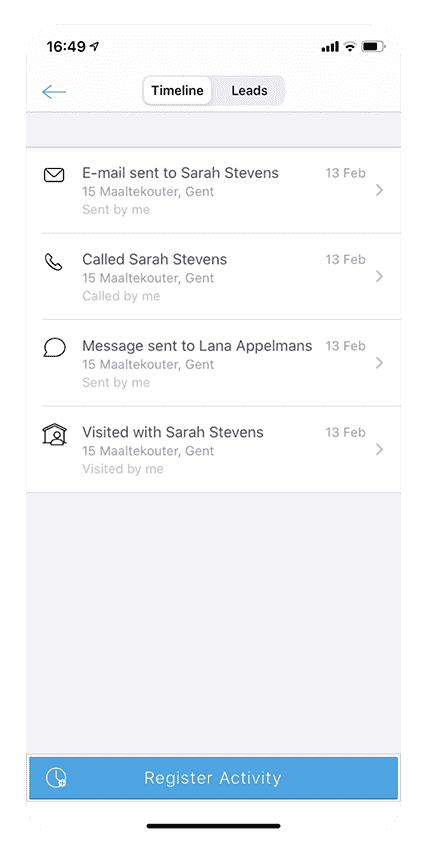The image is a screenshot taken from one phone showing the screen of another phone. The display is set to 16:49 military time. The plane icon indicates the phone is in airplane mode. The status bar shows full cellular signal and Wi-Fi with two bars. The battery is at 75%. 

At the top of the screen, there are navigation controls with a back button on the left and tabs for "Timeline" and "Leads" on the right. The "Timeline" tab is currently active, highlighted with a white background and black lettering, whereas the "Leads" tab is inactive with a gray background and black lettering. 

Below these tabs is a thin horizontal gray divider. The main section displays recent activities, formatted as follows:

- Email sent to Sarah Stevens on February 13th.
  - Sender: Malcolm Turd Gantt
- Call made to Sarah Stevens on February 13th.
  - Caller: Malcolm Turd Gantt
- Message sent to Lana Appleman on February 13th.
  - Sender: Malcolm Turd Gantt
- Visit with Sarah Stevens on February 13th.
  - Visitor: Malcolm Turd Gantt

At the bottom left, there's a clock icon outlined in white against a blue background. Next to it is a button labeled "Register Activity". Above this button sits a large gray box, currently empty. The entire interface appears to be part of a tracking system used for recording interactions such as calls, messages, and visits.